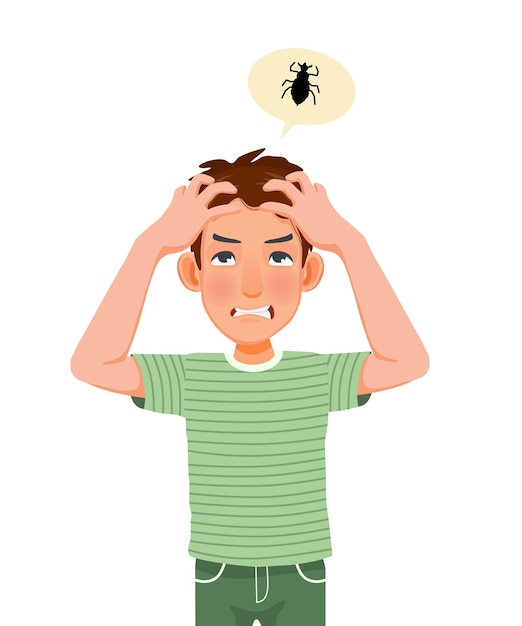The image is a detailed cartoon drawing of a young Caucasian boy, around 10 to 12 years old, with pale pink skin and brown hair. The boy has a concerned, strained expression on his face, gritting his teeth and looking upwards. Both of his hands are buried in his hair as if he's scratching his head. He is wearing a green and black striped short-sleeve polo shirt paired with green jeans that have white lines on them. Above his head is a beige off-white thought bubble containing a detailed black insect, likely symbolizing lice, with six legs, a pointed back end, and pinchers. The illustration captures his distress and confusion, possibly implying he's dealing with lice or similar pests.